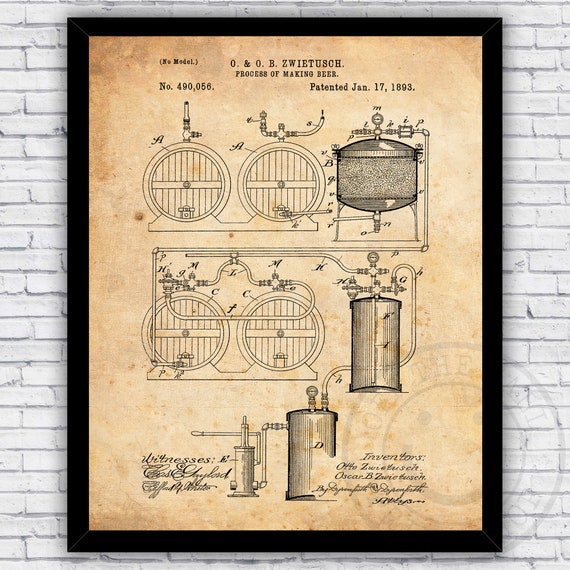The image depicts a framed diagram set against a white brick wall, likely portraying important historical or technical information. The black-framed diagram, drawn on aged brownish parchment paper, outlines the "Process of Making Beer." At the top, it features the label "O&OB" followed by the name "Zwietusch." Prominent in the diagram are several interconnected mechanisms and barrels: at the top left, there are two barrels connected to a mechanism by various tubes, followed by additional barrels and varied apparatuses depicted in subsequent rows. Though some text on the diagram is difficult to read, the detailed illustration provides insight into the step-by-step process involved in beer production. The parchment bears some watermarks near the bottom left, resembling a smiley face with text around it, adding a distinct characteristic to the piece.